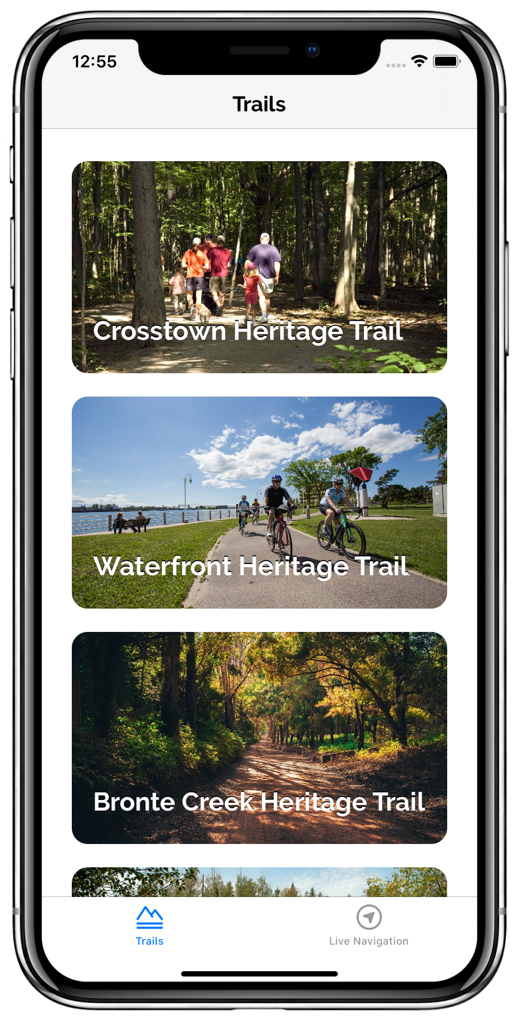**Screenshot of a Trail App**

In this detailed screenshot of a trail app displayed on a smartphone, various trail options are presented, each accompanied by a vivid image and descriptive text. Located at the top left of the screen, the time is shown as 12:55, while the top right displays a nearly full battery indicator.

The app header reads "Trails," and below it, several trail names are listed alongside their respective images. The text is rendered in white, contrasting with the full-color images.

1. **Crosstown Heritage Trail:**
   The topmost option shows a picturesque trail shaded by towering trees, with sporadic sunrays illuminating the path. A family or group of people walks down this serene, leafy trail.

2. **Waterfront Heritage Trail:**
   This option features a scenic trail alongside a waterfront. Here, the ocean is visible on the left, and there are numerous cyclists and joggers enjoying the sunny, clear weather. Trees are sparse, creating an open and airy atmosphere.

3. **Front Creek Heritage Trail:**
   At the bottom, this trail is depicted in an enchanting autumn scene. The path is surrounded by colorful flowers and trees, embodying the beauty of the season.

This app offers a variety of trails, catering to different preferences and showcasing beautiful, natural landscapes.